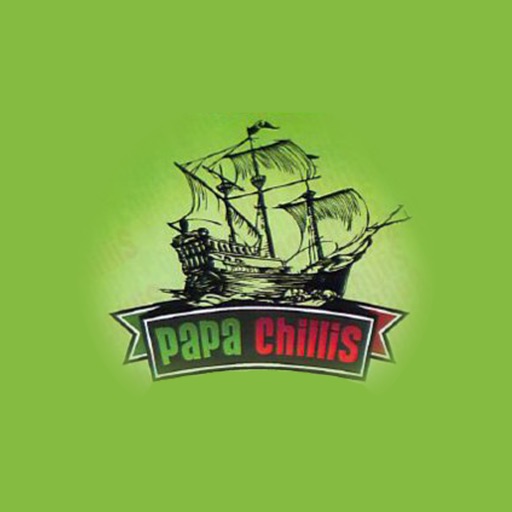In this image, there is a light lime green background featuring a central graphic of a wooden pirate ship, reminiscent of a Spanish galleon from the 1600s or 1700s. The ship, which has three sails and a flag on one pole, appears to be facing to the right and is detailed with a black-and-white, hand-drawn style. The sails are depicted as torn, adding to the vintage pirate ship aesthetic. Below the ship, there is a black and white ribbon banner displaying the words "Papa Chili's" in a distinctive font: "Papa" in green and "Chili's" in red. This likely serves as a logo or advertisement for something labeled "Papachillies" (P-A-P-A-C-H-I-L-L-I-S), integrating both artistic and textual elements seamlessly against the simple, light lime green backdrop.